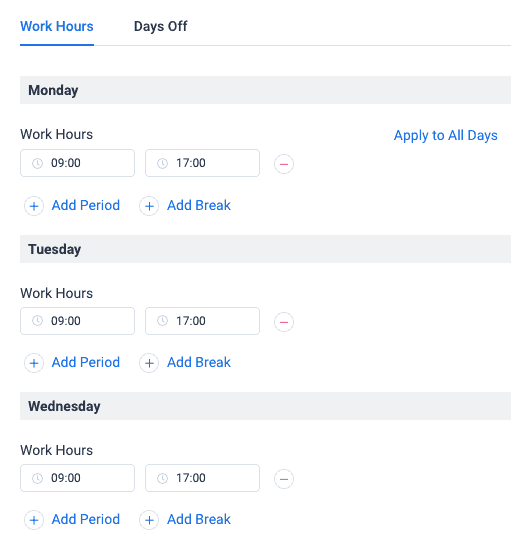This screenshot displays a section of a website or app dedicated to setting work hours and days off, against a pure white background. 

In the top left corner, the options "Work Hours" and "Days Off" are displayed, with "Work Hours" highlighted in blue and underlined, while "Days Off" is in black font. Below this header, there is a white-background menu designed for managing daily work schedules.

At the top of this menu, there's a gray rectangle labeled "Monday" in bold black font. Directly beneath it, in standard black font, it says "Work Hours," followed by two input boxes where users can enter their start and stop times. In this example, the times displayed are 9 to 17. 

In the upper right corner of this section, there's an "Apply to All Days" option. Below the time boxes, there are two blue plus signs labeled "Add Period" and "Add Break." A similar layout follows for subsequent days of the week, such as "Tuesday" and "Wednesday," each with a gray header, input fields for work hours (set to 9 to 17 in this instance), and the options to "Add Period" and "Add Break."

This section allows users to configure their daily work hours comprehensively, ensuring a structured schedule.